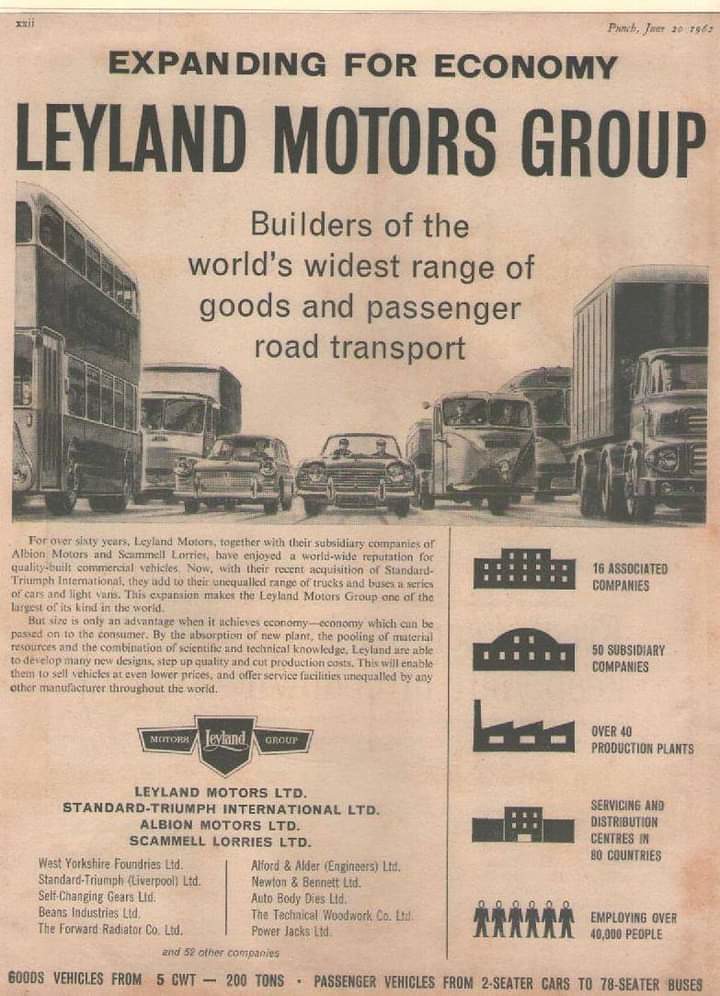The image is a tall, rectangular advertisement resembling an old newspaper or catalogue cover, printed on a burnt off-white or pinkish background. At the top, in bold black text, it reads: "Expanding for Economy, Leland Motors Group." Beneath that, the text states: "Builders of the World's Widest Range of Goods and Passenger Road Transport." Below this heading is a detailed black and white drawing, depicting several lanes of a highway with various cars, buses, and trucks progressing forward. To the left of the image, there's a faded, yet legible column featuring multiple symbols and key statistics about the company: "16 associated companies, 50 subsidiary companies, over 40 production plants, service and distribution centers in 80 countries, employing over 40,000 people." Additionally, in smaller text below the main drawing, it mentions: "For over 60 years, Leland Motors together with their subsidiary companies of Albion Motors and Samuel Loris have enjoyed a worldwide reputation for quality-built commercial vehicles." Details like numbers and addresses are present but too small to read clearly.